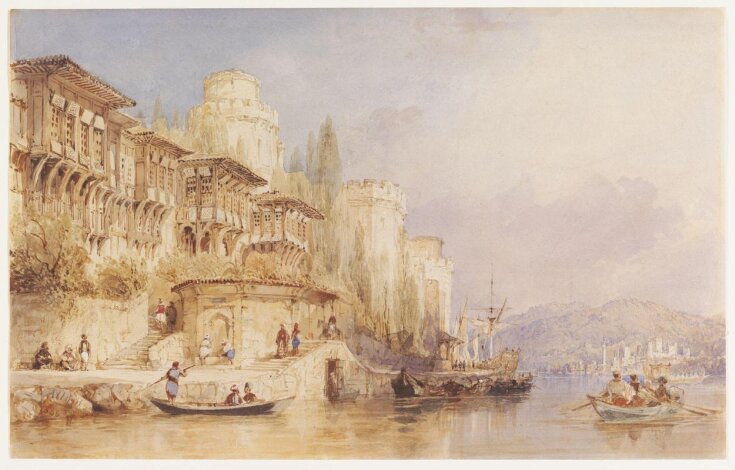The image depicts a large, cream-colored tower with hints of brown, nestled among various other tower-like structures that resemble castles. These buildings, evocative of an ancient city, possibly in Greece or Italy, feature stone steps and white facades that blend seamlessly into a hazy, muted background. The right side of the image reveals a river where gondolas are being rowed by numerous people, adding a lively but serene touch to the scene. The painting, with its muted whites and tans, suggests an Impressionist style but maintains a detailed, Victorian-era aesthetic, possibly evoking a foggy atmosphere that blurs fine details, lending a dreamlike quality to the cityscape.